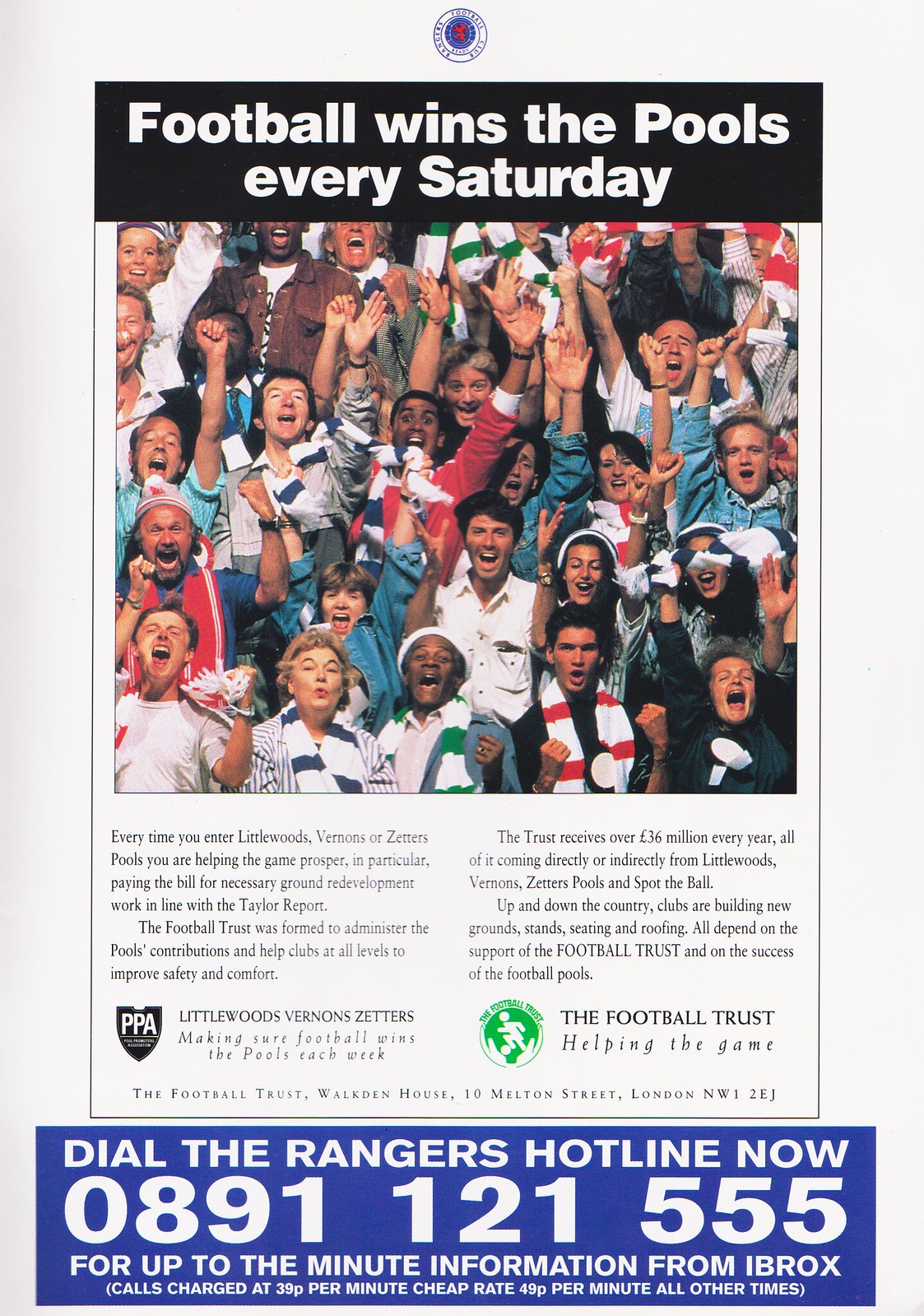The image depicts a page from a soccer program with a light gray background. At the top, a black banner stretches across the page with the white text, "Football wins the pools every Saturday." Beneath the banner, a photograph captures a jubilant crowd of people in the stands, their hands raised and faces beaming with excitement and joy.

Below the photograph, the text explains how participating in Littlewoods, Vernon's, or Zetter's pools contributes to the prosperity of the game by helping to pay for essential ground redevelopment work aligned with the Taylor Report. It goes on to detail that the Football Trust administers these contributions, receiving over £36 million annually from various pools, including Spot the Ball. This funding supports clubs across the country in building new grounds, stands, seating, and roofing, ensuring improved safety and comfort for spectators.

At the bottom of the page, several logos are displayed, including a black badge with "PPA" and a white circle with green text next to "The Football Trust, helping the game." The Football Trust's address, Walden House, 10 Milton Street, London NW1 2EJ, is listed beneath this section. Finally, a red box with white text at the bottom right corner urges readers to dial the Rangers hotline, 0891-121-555, for up-to-the-minute information from Ibrox, with calls charged at 39p per minute during cheap rate times and 49p at other times.